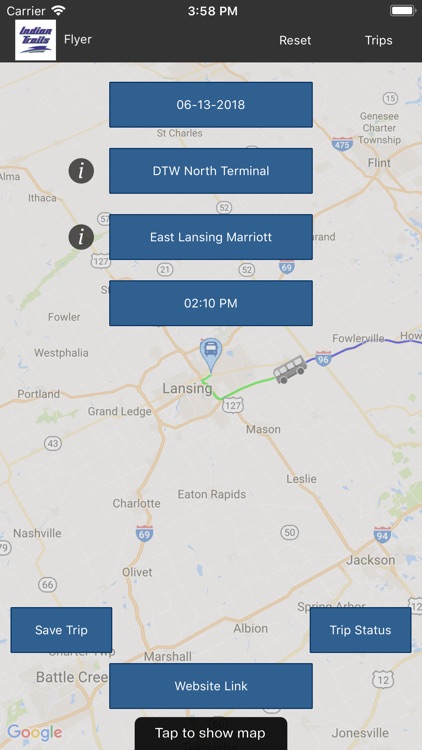A screenshot from a unique version of the Google Maps app displayed on a mobile device showcases a planned trip in Michigan. The map highlights key locations such as Lansing, Eaton Rapids, Jackson, and Flint, signifying it is indeed focused on Michigan. A prominent marker is placed over Lansing. The interface shows several options related to the user's journey, including a timestamp of 2:10 PM on June 13, 2018, with destinations like DTW North Terminal and East Lansing Marriott. 

At the bottom of the screen, there are various buttons: one for saving the trip, another possibly for checking trip status, or accessing a website link. Despite the interface looking unconventional for Google Maps, the recognizable Google logo is visible in the bottom left corner. In the top left, there's a label reading "Indian Trails Flyer," next to reset and trips buttons. Key interstate highways shown include I-94, I-69, and I-96. Additional details reveal a full battery, strong Wi-Fi signal, and the current time as 3:58 PM.